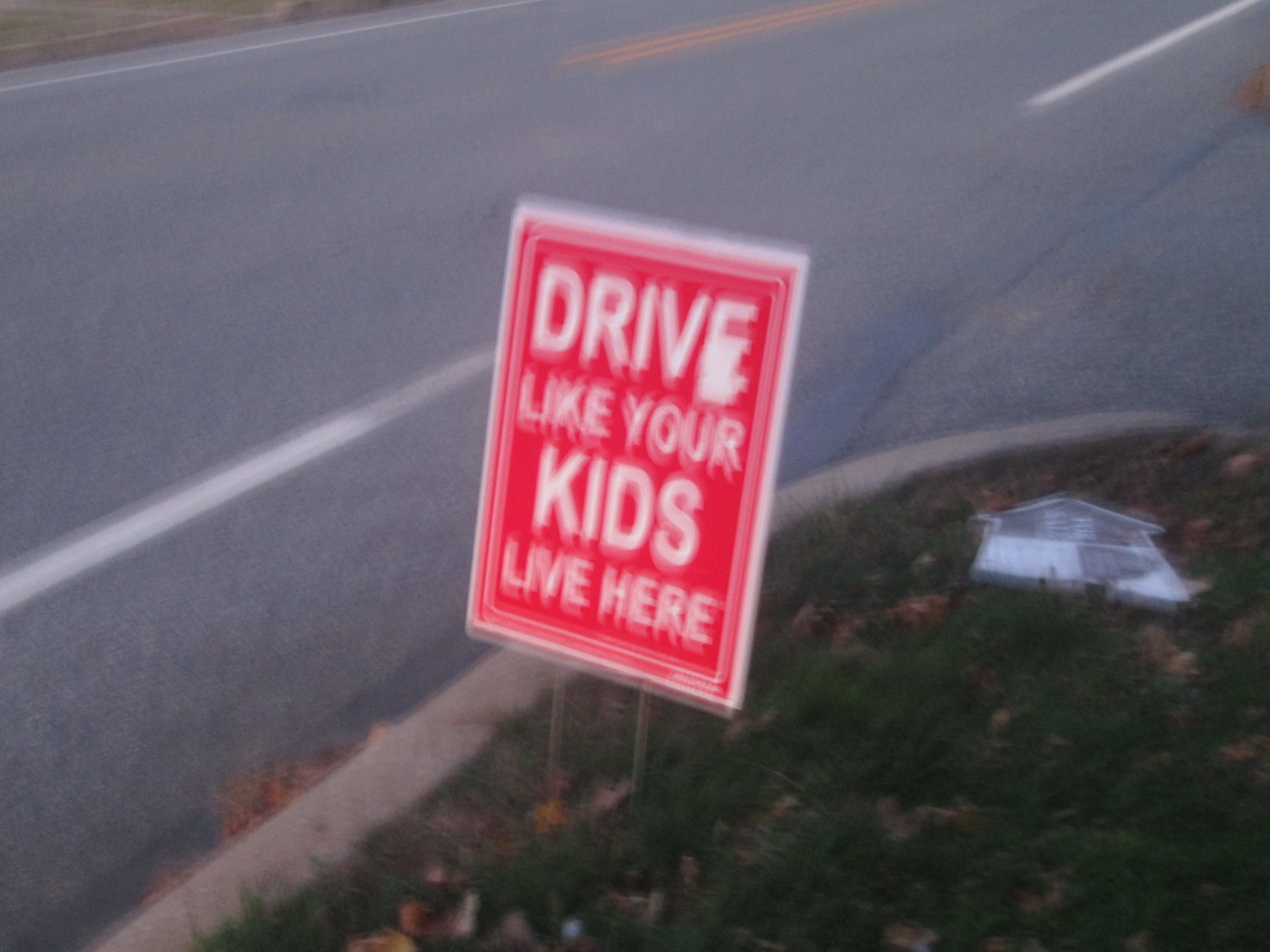The image captures a blurry roadside scene, taken from a low angle, likely while in motion. Dominating the center is a red sign with a white border and white text that reads, "Drive like your kids live here." The sign, supported by two metal spokes, stands on a grassy curb strewn with dead leaves and some litter, including a piece of paper. A fallen white-and-black directional arrow sign is also visible. The grey road in the background features white and double yellow lines, with no people or vehicles in sight.